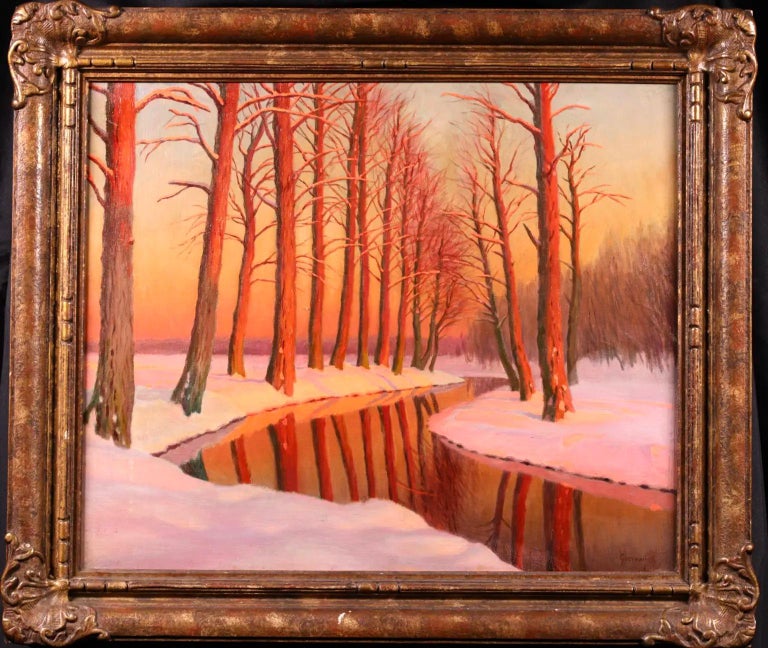This image features a beautifully detailed painting set within a vintage, copper-toned wooden frame adorned with intricate designs at the corners, showcasing signs of age and wear through various shades of browns and reds. The painting itself captures a serene snowy wilderness scene with a gently winding river, which begins at the bottom right and lazily curves through the center. On both banks of the river, tall, bare trees stand stark against the snow-covered ground, their branches devoid of leaves, reflecting majestically in the still water. Further back, we see more trees and possibly rolling hills or mountains under a sky painted with the soft hues of dawn or dusk, transitioning from light blue at the top to warm reds and yellows near the horizon. The painting eloquently conveys the tranquility and cold beauty of a winter landscape bathed in the subtle light of either sunrise or sunset.